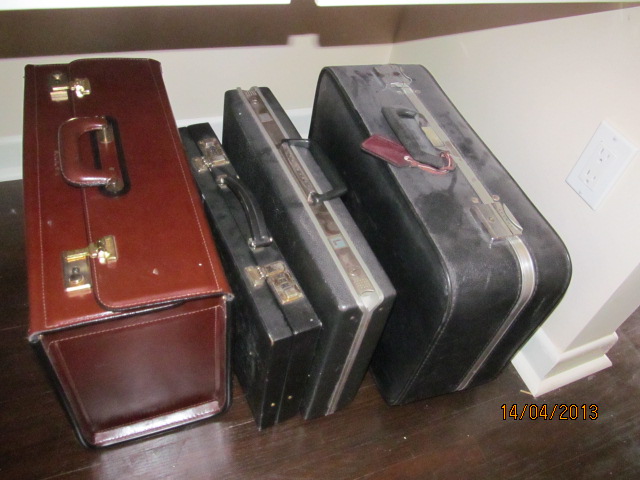In this detailed photograph taken inside a house, dark cherry wood flooring contrasts against pristine white walls adorned with white crown molding along the base. The primary focus is on four briefcases aligned neatly against the edge of a protruding wall on the right-hand side, under a white power outlet. Three of these briefcases are black, dusty, and have black handles with silver clasps and embellishments. The fourth briefcase, on the left, stands out with its clean, dark leather finish, brown handle, and gold clasps, indicating it's better maintained. This leather briefcase also features a distinctive flap that folds over the handle and latches. The photograph, likely a scanned and developed image, is marked with the date "April 14, 2013" in yellow text at the bottom right corner, adding a sense of time to the scene.